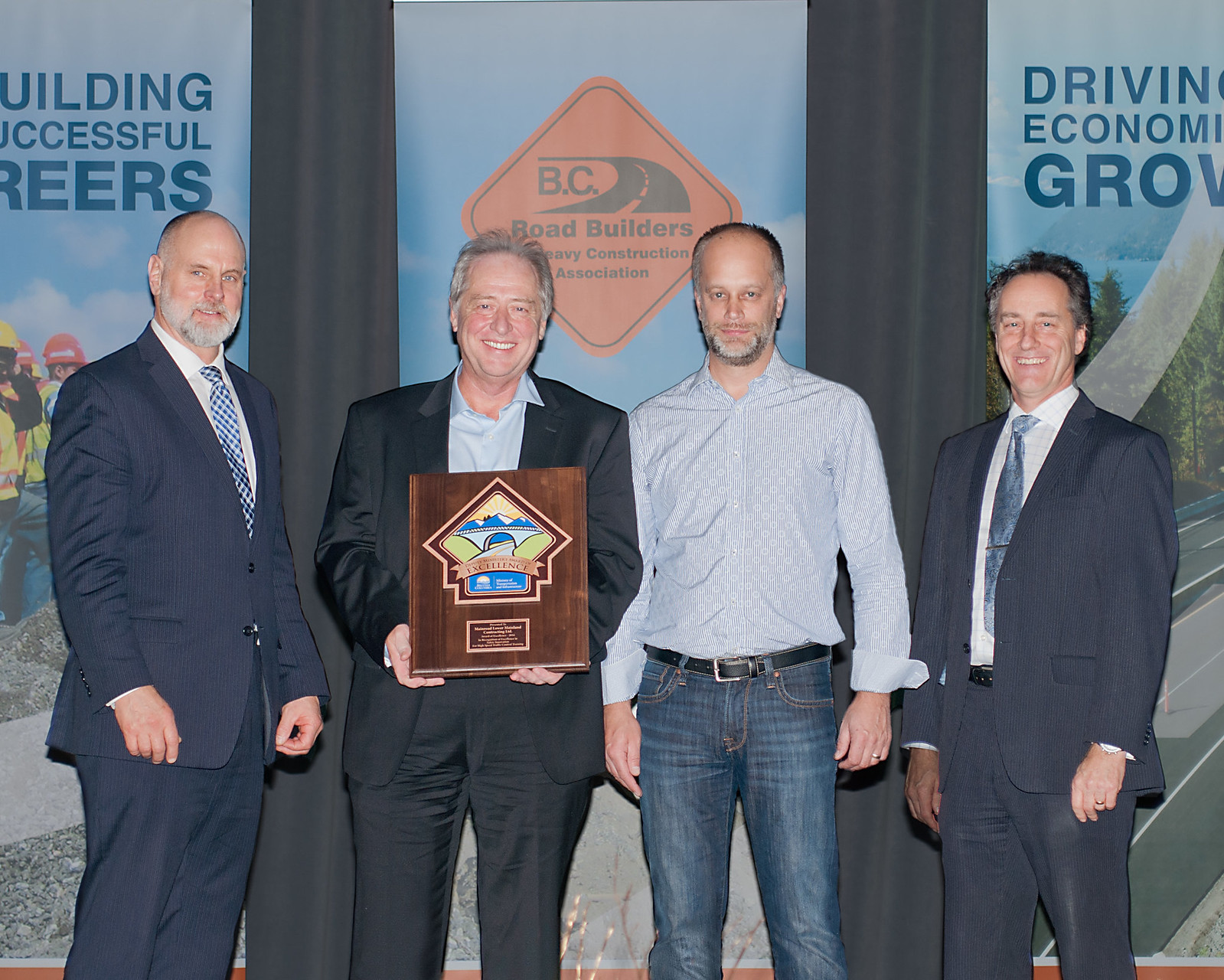The image features four men standing in front of a detailed backdrop. To the far left is a man mostly bald with a white beard, dressed in a dark blue suit and donning a light and dark blue checkered tie. Next to him stands a man holding a brown plaque with blue mountain motifs and the word "Excellence," set against a dark wooden background. He is attired in a black suit with a light undershirt. The man to his right is dressed casually in a light blue button-up shirt with white stripes, blue jeans, and a dark belt; he also has a beard. On the far right is a man in a dark blue suit, a light blue tie, and a white shirt. 

The backdrop presents an orange triangle with "BC Road Builders" written in black, flanked on the left by the words "Building Successful Careers" and on the right by "Driving Economic Growth" in blue letters. Images of roads, trees, and construction workers adorn the background, setting a contextual tone for the event, likely related to construction and infrastructure.